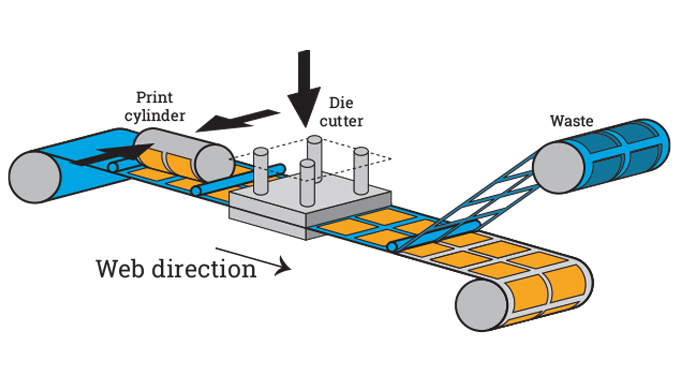The image is a detailed, unlabeled blueprint showcasing a machine involved in a printing and cutting process. Central to the diagram are two primary cylinders: a blue-wrapped Print Cylinder on the left and a gray cylinder on the right. The blue-wrapped cylinder has a blue component extending over its top. Connected via a blue, grid-like pattern, the Print Cylinder is contrasted by the gray cylinder adorned with two yellow boxes on each side and additional yellow boxes beneath it. Between these cylinders is a central square platform identified as the Die Cutter. It features four pegs, each connected to a cylinder at its corners. Arrows point towards the Print Cylinder from both sides, and a downwards arrow targets the Die Cutter platform. Below the Die Cutter, there is an indication labeled Web Direction pointing right. Furthermore, towards the end of the blueprint, there is a blue cylinder labeled Waste, which appears to be rolling up the blue material. The remaining material, now in the form of yellow squares, is collected by another drum, depicting the entire workflow of the machine from printing to waste management.